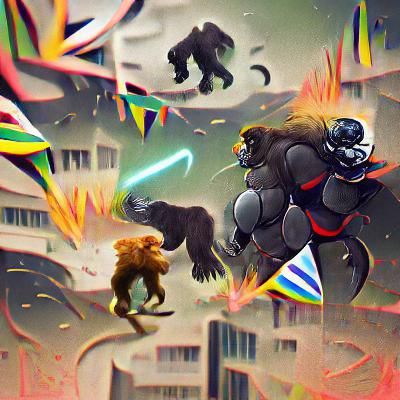The image appears to be a computer-generated scene from a colorful, futuristic video game or graphic artwork, characterized by its square shape and intense visual detail. The central focus is a chaotic battle involving anthropomorphic creatures that resemble armored gorillas or apes, portrayed with intricate, colorful designs. One prominent creature, possibly wearing a clown mask with an orange nose, stands out on the right side, clad in elaborate battle gear. The background features a dramatic landscape of collapsing, fiery buildings in various colors including green, yellow, black, red, and orange, suggestive of mass destruction from some catastrophic event or the ongoing battle. Amidst the chaos, other gorilla-like figures appear to be flying or levitating, contributing to the sense of a high-stakes conflict. The sky is filled with vivid colored stripes and hanging banners, adding to the surreal, animated quality of the scene.